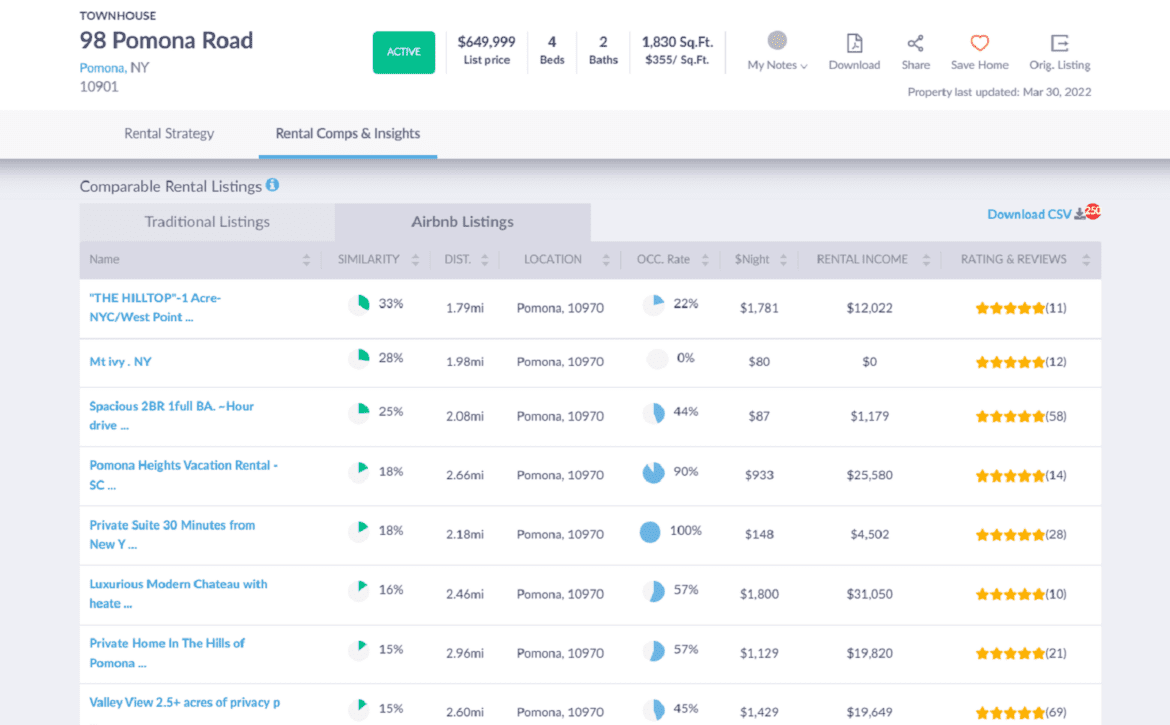For Sale: Stunning Traditional Home in Pomoda - $649,999

This beautifully maintained traditional home in Pomoda features 4 spacious bedrooms and 2 full bathrooms, sprawled across 1,830 square feet of living space. Priced at $350 per square foot, this property offers excellent value with current rental income estimates at $19,000. The home sits on a generous 1-acre lot in the desirable Hilltop neighborhood, providing ample privacy and serene valley views.

The residence was last updated on March 30, 2002, and offers numerous modern amenities, including a luxurious private suite. Perfect for commuters, the property is just a 30-minute drive from New York, and a one-hour drive brings you to Pomoda’s exquisite vacation rentals by the sea.

Enjoy a private home set in the scenic hills of Pomoda, featuring 2.5 acres of complete privacy. Nearby rental comps and property listings indicate strong investment potential, with OCC rates, rental income projections, and a minimum of 5-star ratings adding to its appeal.

All properties in this area, including Valley View and Mt. Ivy, boast an impressive rental occupancy, with Valley View adding up to 20% more at a rate of $1.98. 

Other notable features include a luxurious modern trattoria with heating, making this residence not only a home but a private retreat. Be sure to download the detailed property listing for more information, including rental comparisons, original listing details, and property ratings.

Don’t miss out on this gem in Pomoda - spacious, private, and conveniently located!